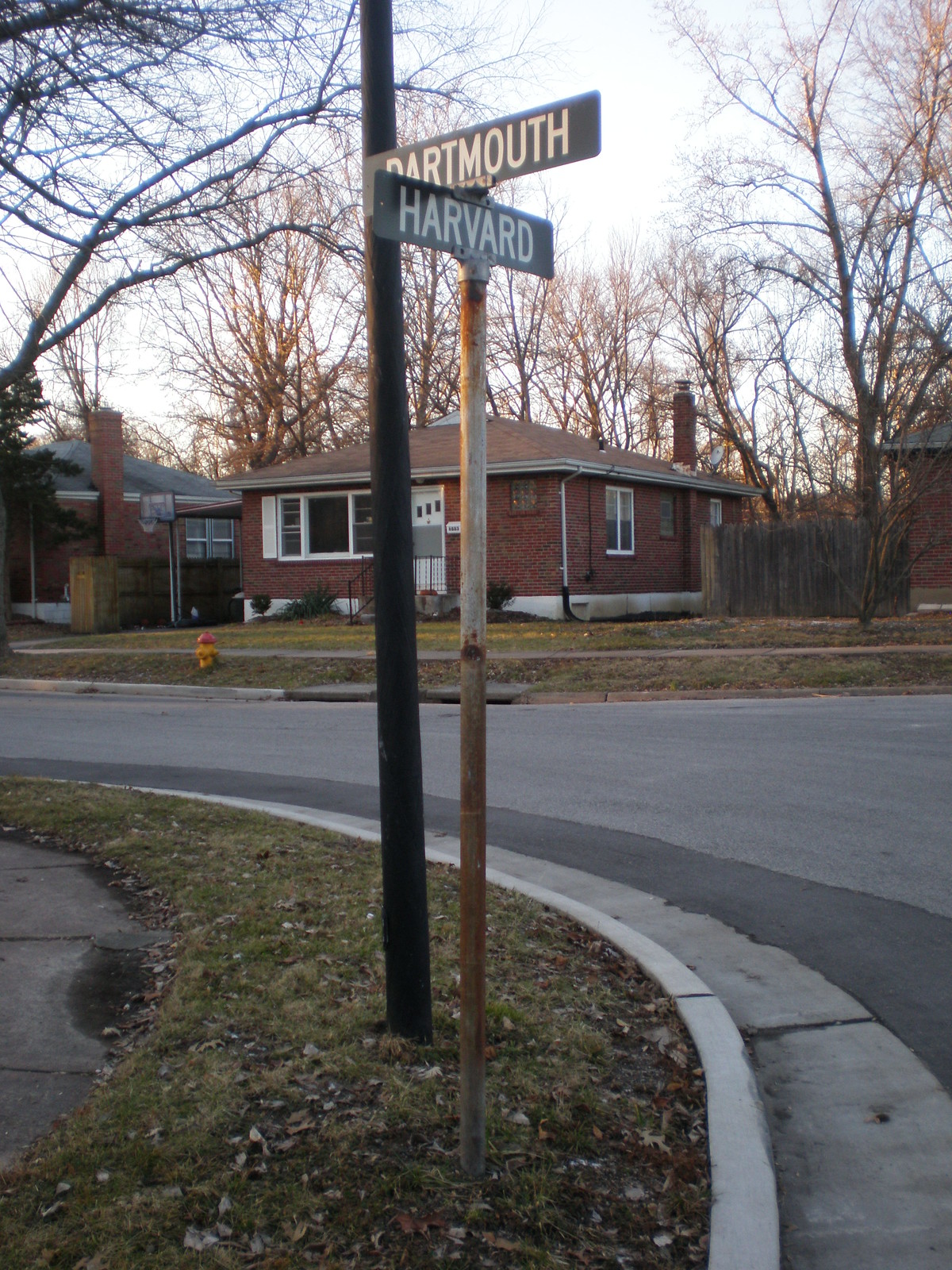A vibrant street corner in a suburban neighborhood captures the viewer's attention with its charming details. At the center of the image, street signs perched on the corner stand prominently, directing traffic and denoting the intersection. The photograph angles upwards, emphasizing the tall signs against the clear sky.

To the left of the image, a well-maintained sidewalk leads the eye past a lush, grassy verge that gently curves with the street corner. The pavement's curve elegantly guides the viewer's gaze towards a peaceful suburban street.

Across the street, a row of inviting brick homes faces toward the camera. The house at the center, featuring a striking white door, stands out as a focal point, contributing to the neighborhood's welcoming atmosphere. The overall composition of the image adeptly combines architectural and natural elements, providing a comprehensive view of this tranquil suburban scene.